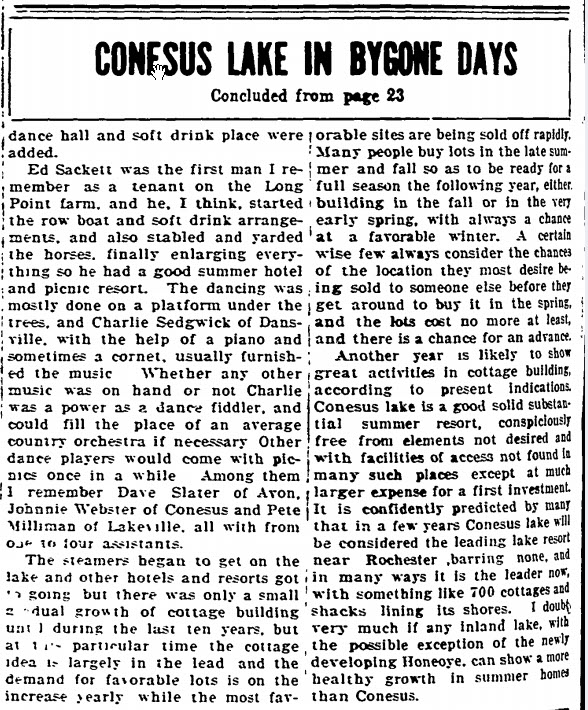The image is a photograph or scan of an old newspaper, primarily black and white in color. The layout features a distinct black-outlined rectangle at the top with the title "Conesus Lake in Bygone Days" written in large, bold, capitalized black font. Beneath this title, in smaller black font, is the note "Concluded from page 23." The page is divided into two densely packed columns of text filling the remaining space. The article starts mid-sentence and continues with a narrative about a man named Ed Sackett, who pioneered various leisure activities at Long Point Farm, eventually developing it into a summer hotel and picnic resort. Additional text details events like platform dancing under trees, with music provided by Charlie Sedgwick of Dansville, involving a piano and sometimes a cornet. The entire image gives the impression of an old, possibly photocopied, text excerpt. A noticeable detail is the small hand-shaped cursor pointer in the image, adding a modern digital layer to the otherwise historical setting.